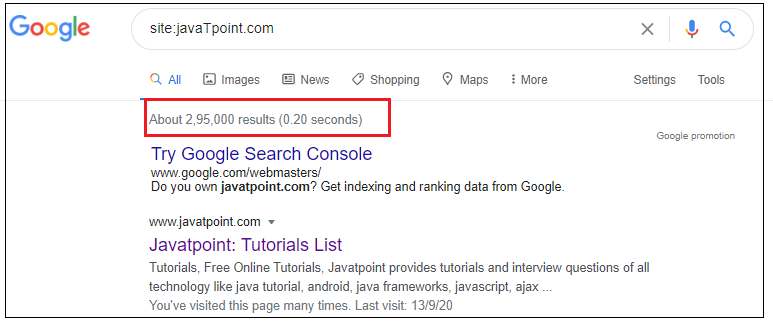The top portion of the image features the Google logo prominently on the left-hand side, with each letter in its signature colors: the first letter 'G' is blue, 'o' is red, 'o' is yellow, 'g' is blue, 'l' is green, and 'e' is red. Below the logo is an oval search box with a gray outline. Inside the box, text in black reads "site.dravotpoint.com". To the right of the search box is a gray 'X', followed by a vertical line, and then a blue microphone icon alongside a white magnifying glass icon.

Below the search bar, the text "All" is highlighted in blue, while other text options including "Images", "News", "Shopping", "Maps", and "More" are in black. On the left side, there are three circles, and additional options "Settings" and "Tools" are also present.

Within a red box, it displays, "About 295,000 results (0.20 seconds)" in black text. Following this, text in blue reads "Try Google Search Console", while below that, black text states, "www.google.com/webmaster/do you own dravotpoint.com? Get indexing and ranking data from google.com."

In the main body of the results, the first link, "www.javatpoint.com", is displayed in black, followed by, "javatpoint.com tutorials list" in purple. The description underneath, in black text, mentions "Tutorial suite, online tutorials, Javatpoint provides tutorials and interview questions on all technologies like Java tutorial, Android, Java frameworks, JavaScript, AJAX,..."